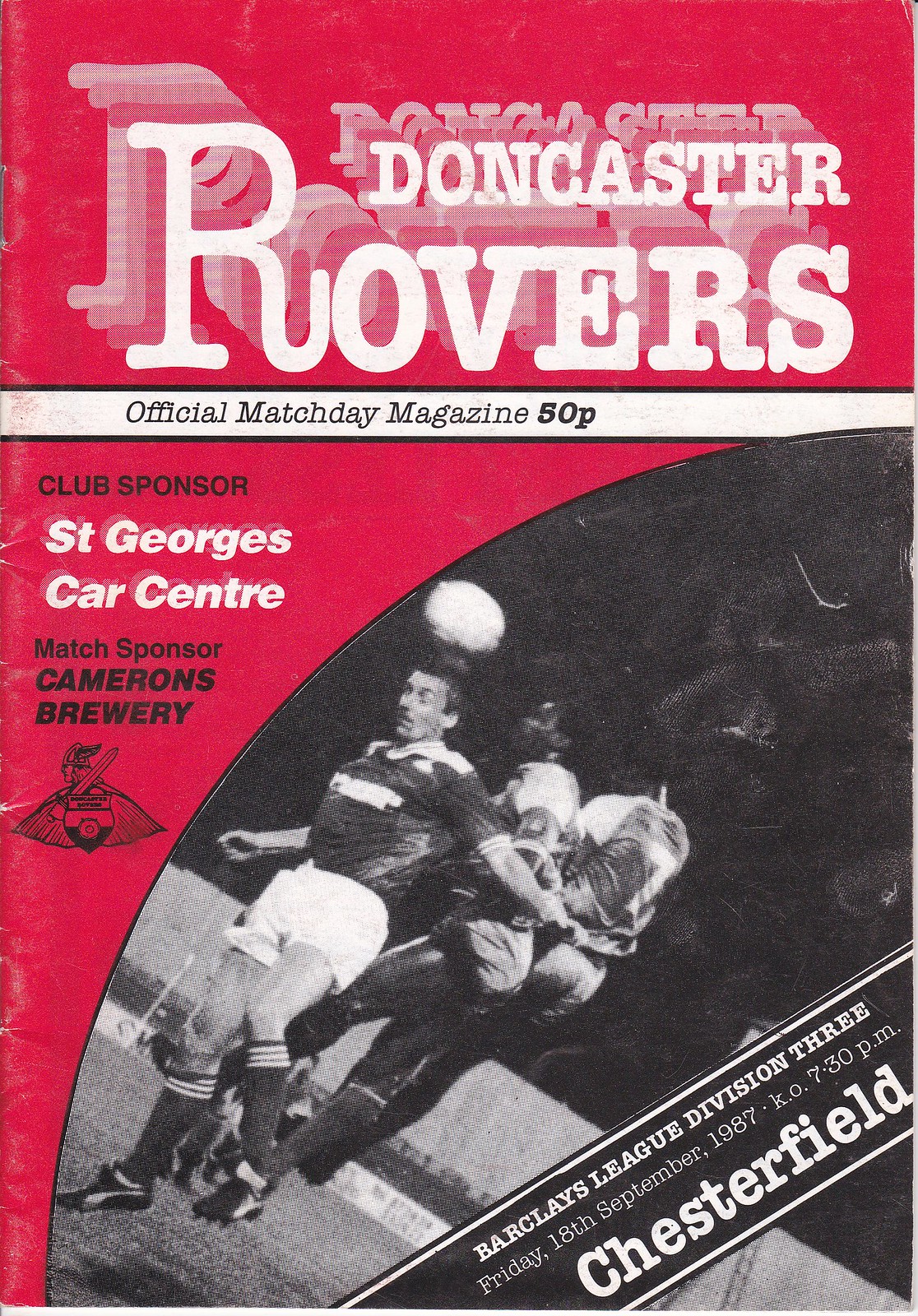This is a vertical rectangular image resembling a magazine cover for the Doncaster Rovers soccer club. At the top, in large white letters with shadows creating a graduated effect, it reads "Doncaster Rovers" against a red background. Beneath it, a white band stretches across with black text stating "official match day magazine" and the price, "50 pence."

Further down, additional sponsor information appears. "Club sponsor" is written in red against the red background, followed by "St. George's Car Center" in white print. Below this, "Match sponsor Cameron's Bakery" is written in black, accompanied by the bakery's symbol.

The lower section of the cover features an action photograph from a soccer match. In the image, a player with a dark jersey and white shorts heads the ball, while two other players—one in a white jersey with dark shorts and another partially visible—are nearby. To the right, a vertical black banner with white text states, "Barclays League Division 3, Friday 18th September 1987, Kickoff 7:30 p.m." Below this, in large white letters, "Chesterfield" is written. The overall design captures both the dynamic action of the game and essential match details.